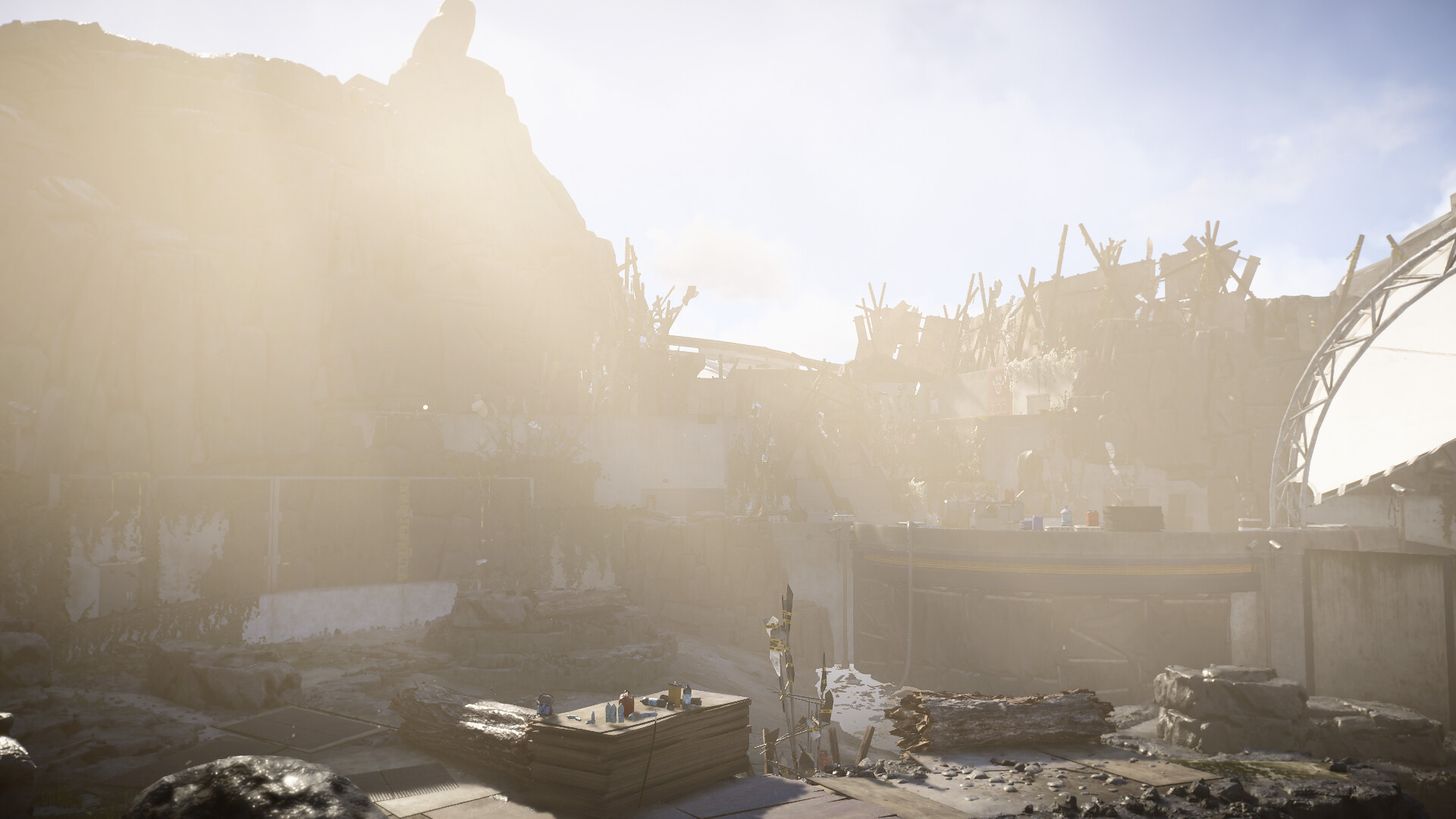In this computer-generated image, a partially collapsed bridge dominates the scene, evoking a post-apocalyptic atmosphere. The bridge, possibly once grand, now lies in ruins with fragments of cement and twisted metal beams jutting out at odd angles. Above, a clear blue sky offers contrast to the decaying structure, although a hazy layer of brownish sunlight or dust bathes the landscape, adding to the desolate feel. 

A broken tree, its splinters visibly protruding, stands as a silent witness to the chaos. In the center of the image, pieces of lumber are scattered, with what appears to be cups haphazardly placed atop them. To the right, a yellow stripe marks one of the remaining cement embankments, indicating its original structural importance.

Overall, the scene suggests a once-functional bridge now overtaken by time and decay, rendered with a level of detail that hints at its origin in a video game or fantasy movie, capturing a unique and eerie beauty in its desolation.